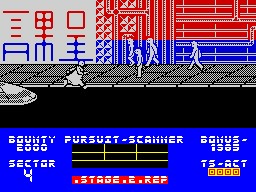This image depicts a vintage video game scene with rudimentary, low-resolution graphics. The primary focus is a dark, narrow street flanked by a grey sidewalk, populated by white figures outlined in black. The urban backdrop features buildings shaded in hues of red, black, and grey, enhancing the sense of a bustling cityscape. To the left side of the street, there appears to be a crudely rendered vehicle. The bottom quarter of the image is dominated by a blue overlay displaying game information, albeit in a highly pixelated and barely legible font. Phrases such as "Pursuit," "Scanner," or possibly "Scammer," along with "Sector 4" are faintly discernible, hinting at the in-game objectives or level identifiers. The overall graphical quality is notably poor, characteristic of early video game design.